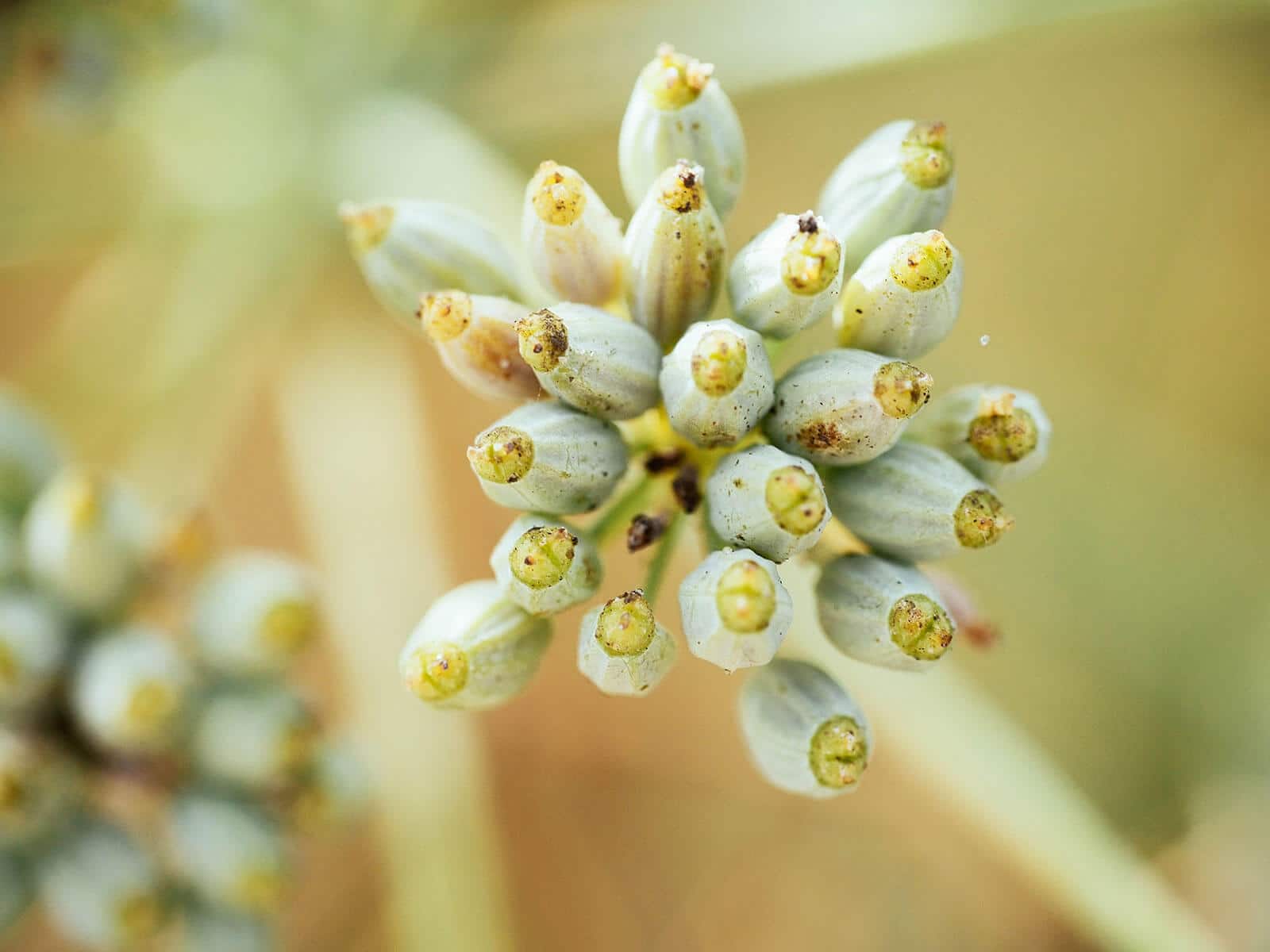This macro shot highlights an unbloomed desert plant with a distinct close-up of its buds. The cluster features buds shaped like footballs or olives, predominantly light green with hues of yellow, white, and hints of orange. Each bud has a yellow circular tip, possibly indicating the flower's center, and a subtle corrugated texture, suggesting their immature stage. The buds are aligned, protruding uniformly from the cluster. Blurred, earthy background tones of tan, light green, and white emphasize the focus on the cluster, with the stalk and additional buds in the lower left also out of focus. The background includes an indistinct green element, adding depth to the image. Tiny specks, likely pollen, coat the buds, enhancing their detailed appearance.